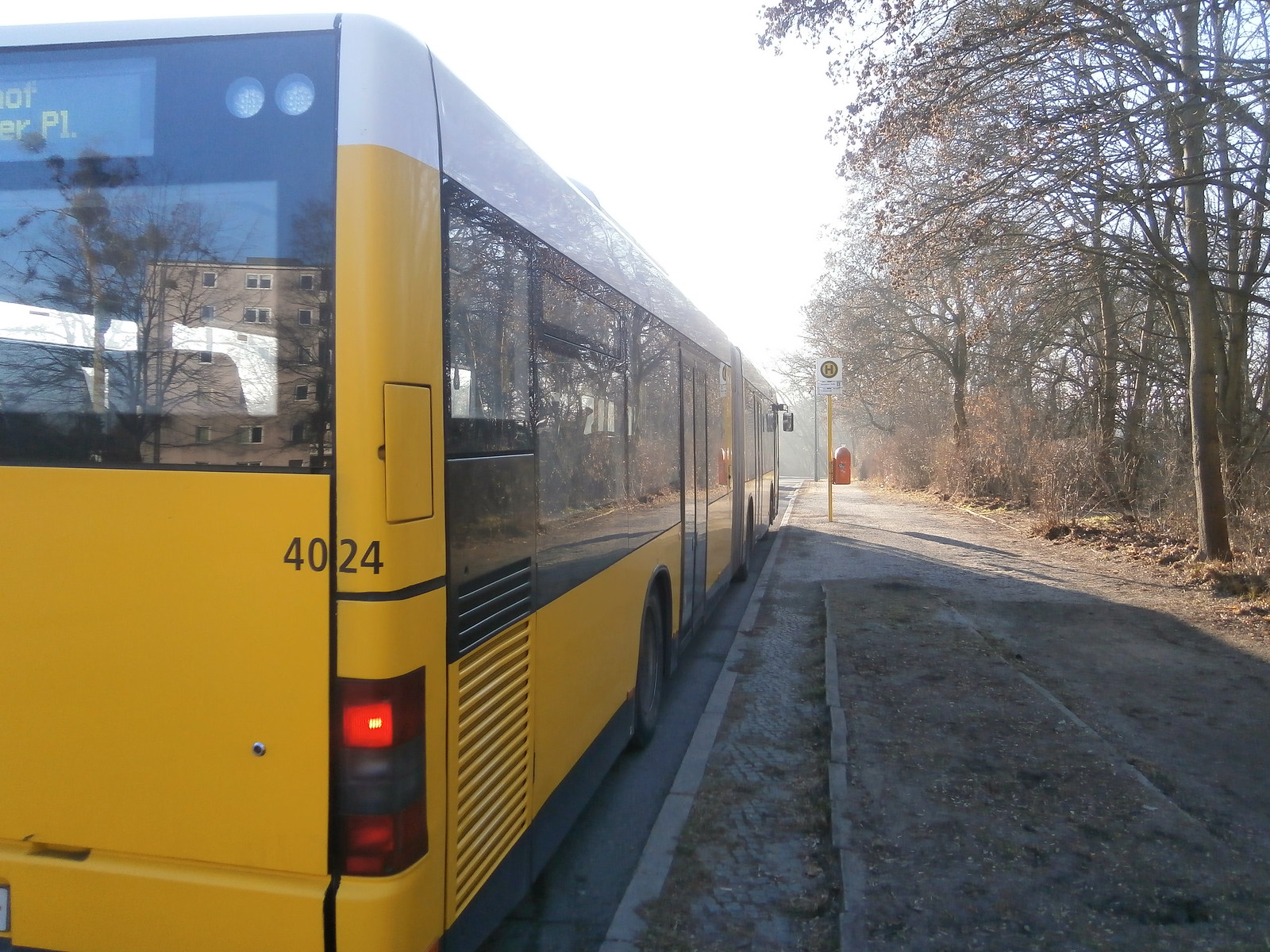This outdoor photograph captures the rear view of a distinct, elongated yellow bus, identified as bus number 4024. The bus, resembling the style of an accordion or articulated bus commonly seen in city transit systems, features a blocky, double-length structure with accordion material in the middle allowing it to navigate corners. Its yellow body is complemented by a white panel running along the top, clear windows outlined in black metal, and a white roof. The scene is framed by a dirt sidewalk and a path, running alongside dense, leaf-bare trees indicative of winter or late autumn. The curbside bus stop is marked by a yellow pole with a white sign displaying an H in a yellow, black-outlined circle, and a small box attached to the pole, potentially a trash bin. Reflections in the bus's rear windows reveal a brick building, and the windows also allow a view through to trees on the opposite side of the road. The brake lights are lit red, adding to the detailed portrayal of the setting.